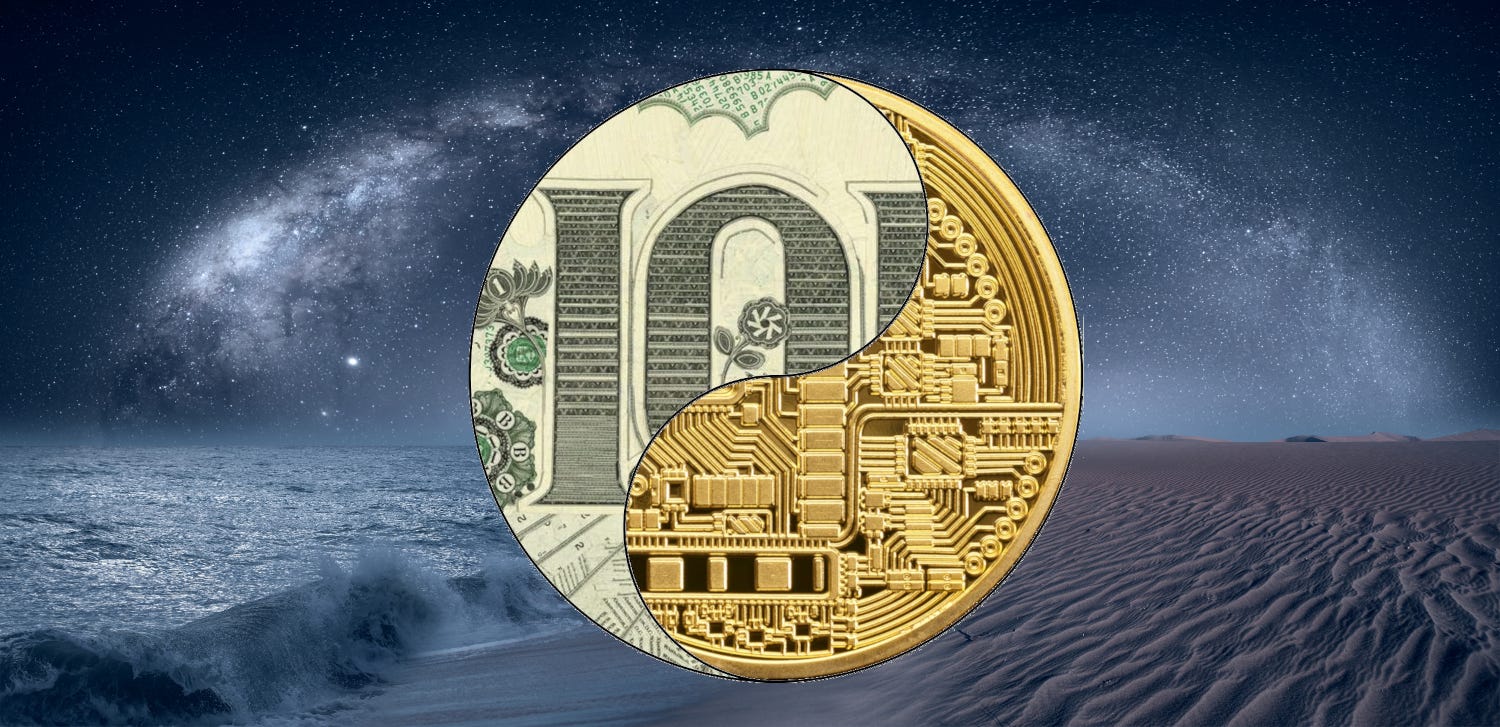This computer-generated illustration showcases a circular design with a yin-yang pattern at its core. In the top left portion of the circle, there's a detailed segment of a $100 bill, recognizable by the visible "$100" and surrounding symbols, rendered in green and white. The bottom right portion contrasts with a depiction of a computer circuit board, featuring intricate gold-plated circuits that convey a sense of technological depth.

The background is split into two contrasting landscapes: to the left, ocean waves crash against a beach, while to the right, desert sands stretch under the vast night sky. Above these scenes, a star-filled sky, reminiscent of the Milky Way, envelops the entire composition, adding a celestial touch to the imagery. This juxtaposition of nature, technology, and currency within a yin-yang framework highlights the interconnectedness and duality of these elements.